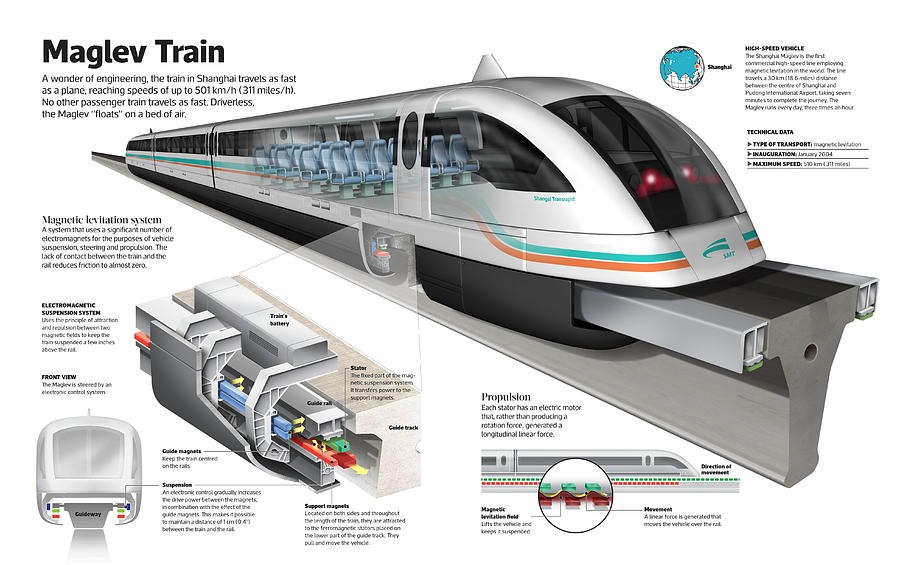This virtual poster is an informative and detailed diagram of the Maglev train, renowned as a wonder of engineering. Located in the top-left corner is the title "Maglev Train" followed by the tagline, "a wonder of engineering." Below that, the poster emphasizes that the Maglev train in Shanghai travels as fast as a plane, reaching speeds of up to 501 kilometers per hour (311 miles per hour), making it the fastest passenger train in the world. Notably, this driverless train floats on a bed of air through magnetic levitation.

The central portion of the poster features an image of the sleek, bright silver Maglev train, adorned with decals of cyan and orange stripes. Surrounding the train image are various diagrams and close-up views that demonstrate and describe its different components, including its magnetic levitation system and propulsion mechanism. To the right of the main train image is a photograph of the train itself, while above this section sits a globe pinpointing Shanghai.

The diagram is further annotated with numerous descriptions and exploded views, illustrating how the Maglev's different parts function, thereby offering a comprehensive understanding of this high-speed marvel of modern transportation.